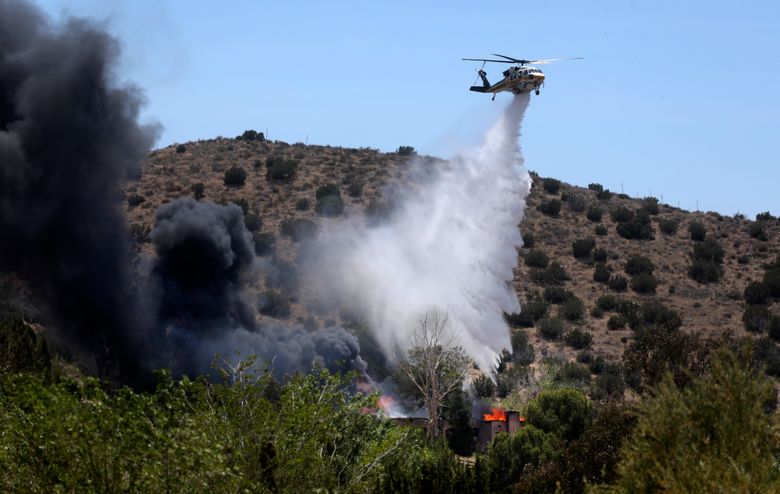In the image, a helicopter is seen hovering in a bright, blue sky, diligently dropping water to extinguish a forest fire. The flames are causing black smoke to rise high into the air from a burning, dried hillside typical of California terrain, dotted with the occasional bush and some green trees. The area is a mix of charred land and patches of dead grass, with a backdrop of brown, rugged mountains. On the left side, thick, dark smoke billows heavily, while on the right, the helicopter releases a torrent of water aimed at dousing the persistent flames and calming the fire. The landscape shows signs of severe burning, with little flames and embers still visible amidst the damaged foliage. Some houses can be faintly seen in the distance, highlighting the urgency and importance of the firefighting effort.